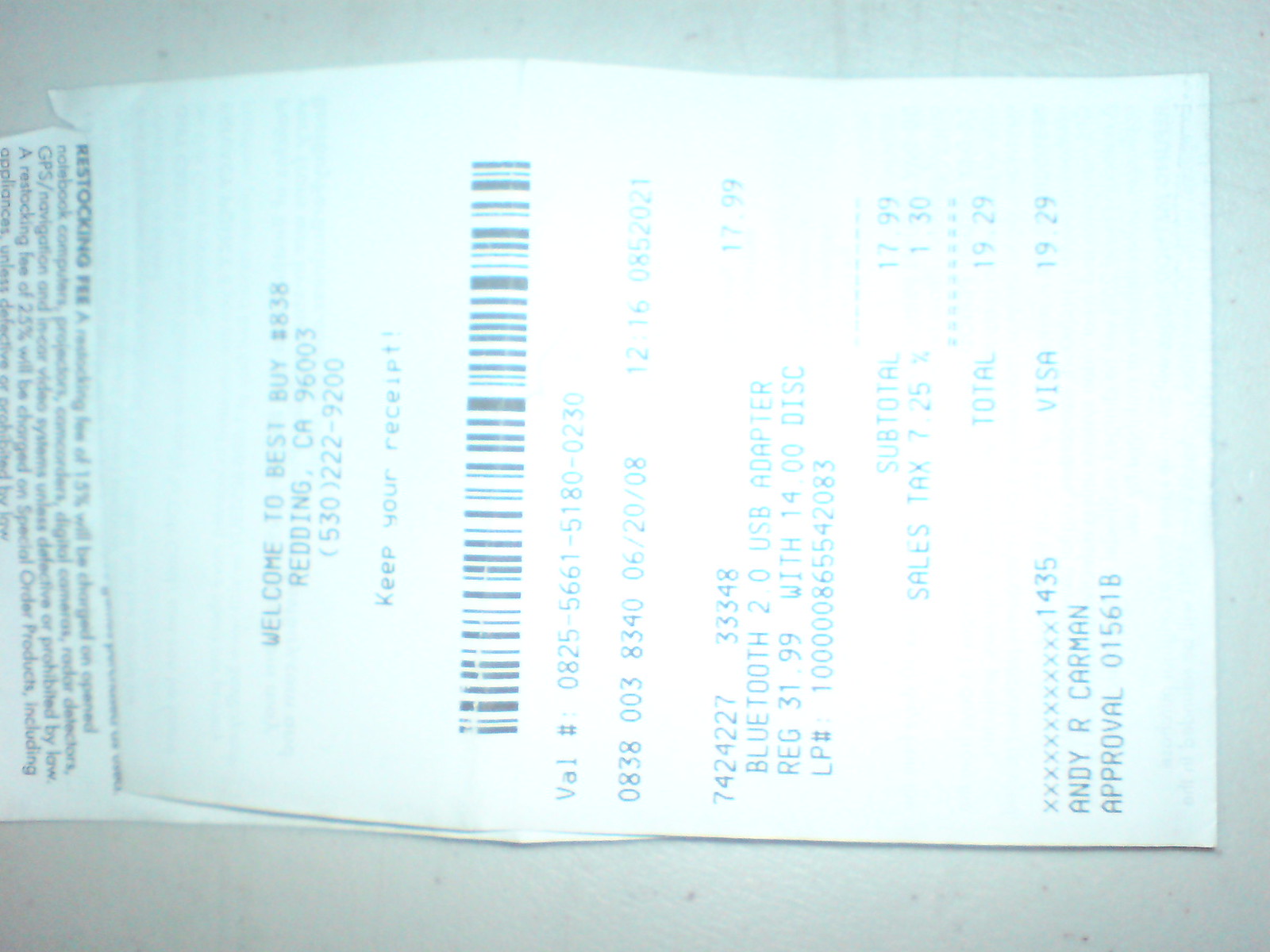The image is a color photograph in a landscape orientation, featuring a folded till receipt from Best Buy. The receipt, printed on thin, slightly glossy paper, lies across the center of the image. Its slight curvature and fold create a gentle arch, with a portion of the receipt extending upwards behind the main section. To properly read the text, the image would need to be rotated 90 degrees clockwise. Despite a reflective highlight—likely from the camera's flash—obscuring some details, the text is mostly legible.

At the top of the receipt, the text reads "Welcome to Best Buy," followed by the store's location: "Reading, CA 96003." Below this, a contact phone number, "530 222 9200," is visible. Further down, the receipt details the total payment, made with a Visa card ending in 1435, which amounted to $19.29. The purchase was for a "Bluetooth 2.0 USB adapter."